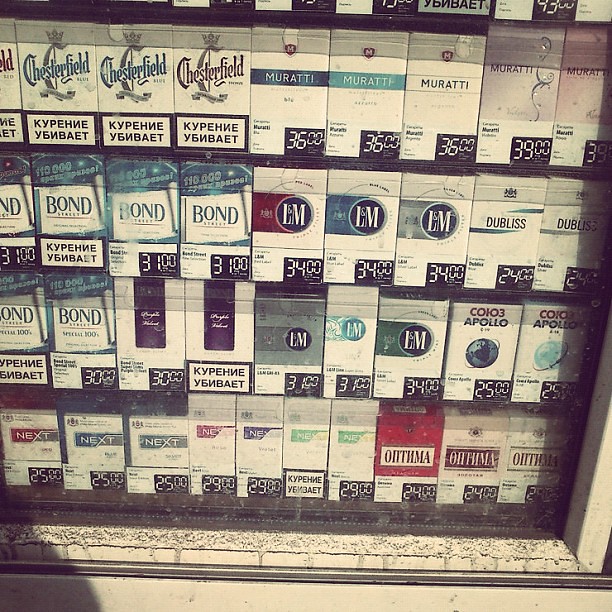The photograph captures a detailed view of a vending machine featuring a large display of cigarettes for sale. Encased behind a glass window with a cement ledge, the display consists of at least four rows, possibly a fifth, each packed with various brands including Chesterfield, Bond, L&M, and others. The cigarette cartons vary in color, predominantly white with accents of blue, red, and green. Clear white or green lettering can be seen on the boxes, some of which are labeled in English while others appear in a Cyrillic script, suggesting they might be Russian. Prices are prominently displayed on the cartons, mostly in the $30 range such as $36 and $31, with a few priced in the $20s. The vending machine itself, made of white metal, shows signs of wear with visible dirt.